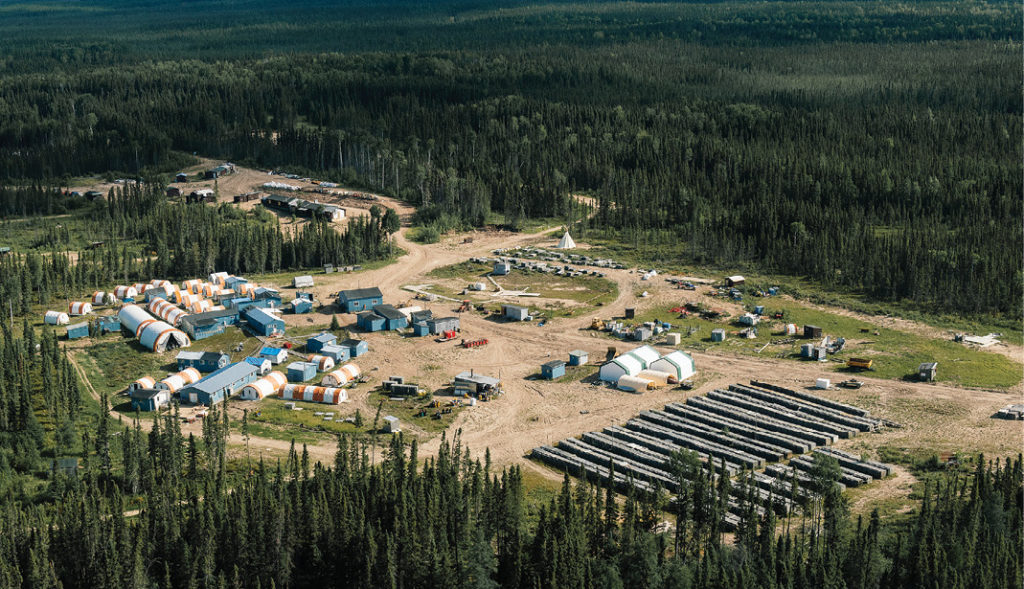This aerial photograph captures a sprawling, secluded farm nestled atop a mountain, surrounded by lush, deep green forests with tree canopies visible in the foreground. The farm features an expansive open lot with several buildings, including barns and one-story structures in shades of white, blue, and cream, all with dark roofs. Long rows of large cylindrical hay bales, wrapped in plastic, are meticulously arranged across the landscape. To the right, there are wooden planks resembling railroad ties, stacked in multiple neat rows. The image gives a detailed view of dirt roads crisscrossing the site and an assortment of small, cylindrical objects scattered across the ground, possibly concrete markers. It seems to be a work site, devoid of people, with elements suggesting both agricultural and manufacturing activities. The overall scene, possibly captured from an airplane or helicopter, exudes an air of serene isolation and natural beauty.